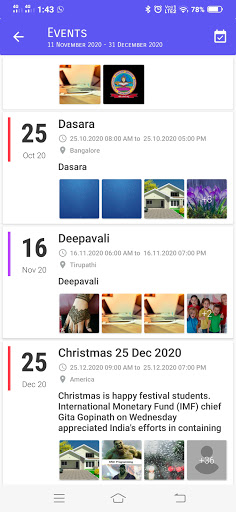This image captures a screenshot of a cell phone display showcasing a calendar or event management app. The top section of the screen is bordered in blue and indicates the time with the number "143" in the top left corner. On the top right corner, various icons including the Bluetooth and battery indicators are visible.

Beneath the top section, there is a navigation bar featuring a left-pointing arrow followed by the word "Events" and the date range "11 November 2020 - 31 December 2020." Alongside this text is an icon of a calendar with a white check mark over it.

The main content area contains two segments of dated events. The first segment displays two images. The left image is highly out of focus with dominant tan colors, possibly depicting a desk or table with several items on it. The adjacent image has a black background featuring a multicolored round symbol. Text beneath this segment states "25 October 2020. Dasara. 25-10-2020. 8 a.m. - 25-10-2020. 5 p.m. Dasara." Below this, there are four square photographs: two are filled with a solid blue color, the third shows a house with a driveway and open garage, and the last picture depicts grass and a purple background with an overlay saying "+8."

Next, the segment dated "16 November 2020" is labeled "Depot Valley" and shows four images. The first image is of a person's hand, but the other two are unclear due to being out of focus. The fourth image is of a group of children gathered together.

Finally, the bottom of the screen details "25 December 2020" with the event "Christmas," accompanied by the words "Christmas is happy festival students." There is an additional textual snippet mentioning "International Monetary Fund chief Gita Gopinath on Wednesday appreciated India's efforts in containing..."

Overall, the image represents a mixture of visual content and text documenting specific events over a timeframe, showcasing both clear and unclear photographic imagery along with indicative timestamps and event descriptions.